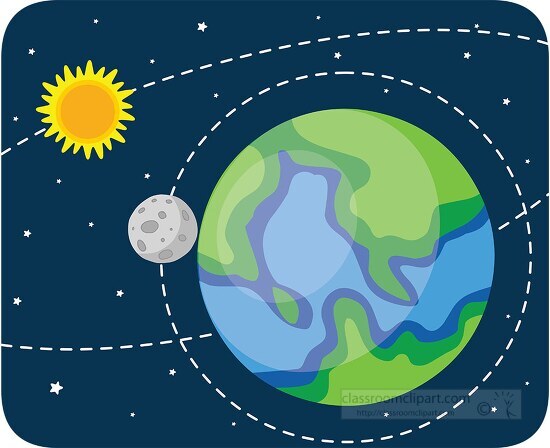The image is a vibrant, cartoonish illustration of the solar system with particular focus on the Earth, the Moon, and the Sun. Set against a navy-blue background adorned with small, hand-drawn white star shapes, the Earth is centrally located towards the bottom right corner, depicted in abstract, splotchy blues and greens. Encircling the Earth is a white, dashed line representing the Moon's orbit. The Moon, gray with darker gray spots, is positioned to the left of the Earth along the dashed orbit line. In the top left corner, the Sun radiates in a bright orange core with cartoonish yellow flares. Another dashed oval line extends from the Sun to indicate the Earth's orbit around it. The bottom right corner of the image features a semi-transparent logo with the text "classroomclipart.com," revealing the source of the clip art graphic.